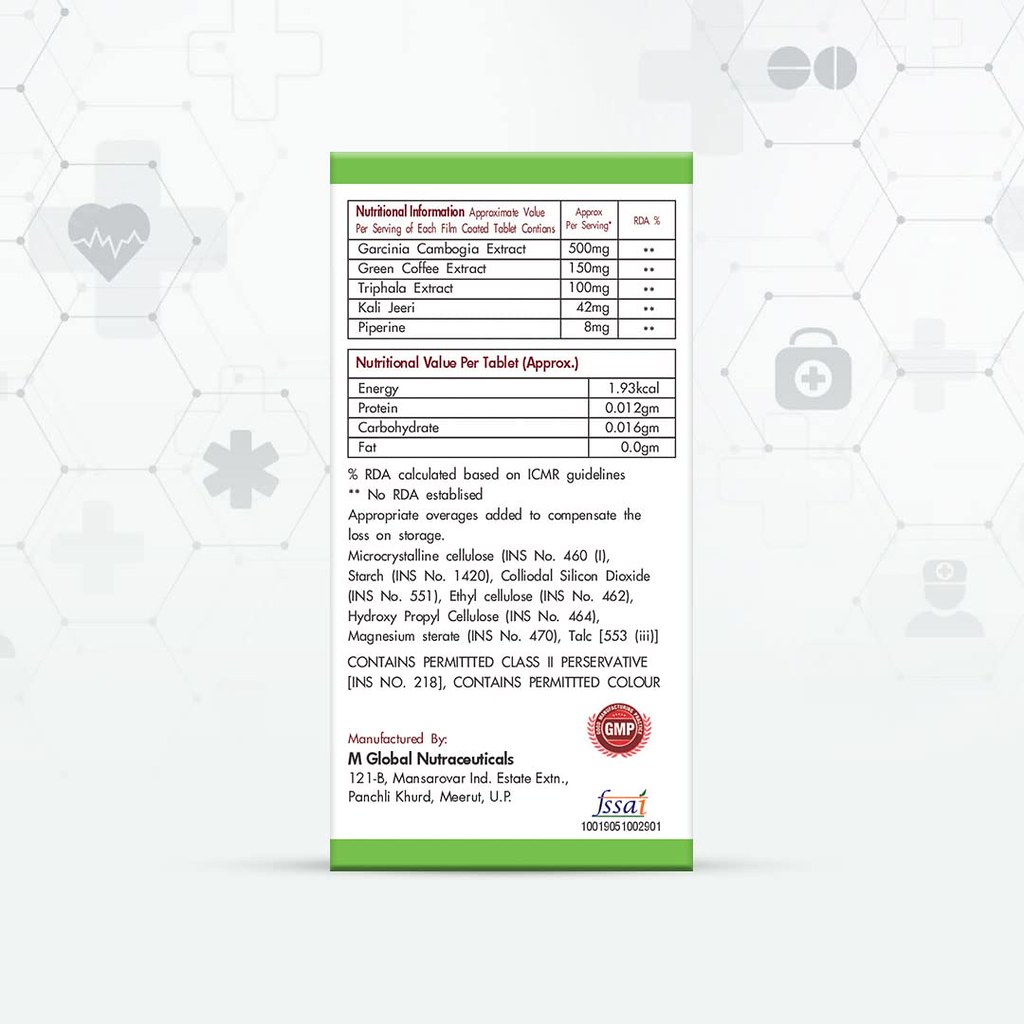This image depicts the side of a white box featuring detailed nutritional information for a dietary supplement manufactured by M-Global Nutraceuticals, located in Panjshir Khurd, Merut, UP, India. The background of the box is light gray with a pattern of hexagons outlined in the same light gray color. Within some of these hexagons, there are various medical-themed icons, such as a heart with an EKG line, a medical star, a first aid kit with a cross, a pair of divided circles, and a doctor icon with a cross on the hat.

At the center of the image, there is a vertical white rectangle bordered by green bands at the top and bottom. This rectangle contains a chart listing the nutritional information, including ingredients like Garcinia cambogia extract with serving size (500 milligrams) and ROA percentage, among other components. Below this chart, another table details the nutritional value per tablet, specifying values for energy (1.93 kcal), protein (0.012 gm), carbohydrate (0.016 gm), and fat (0.0 gm).

Adjacent to these charts, additional text and logos provide more details. On the right side, a red circle with a white 'GMP' label is visible. To the left, the text states "Manufactured by: M Global Nutraceuticals" followed by the address. At the lower right corner, there is an FSSAI logo along with a long identification number beneath it. The label also indicates the presence of other ingredients such as green coffee extract, triphala extract, colligeri, and piperine, with the tablet being described as microcrystalline cellulose-type.